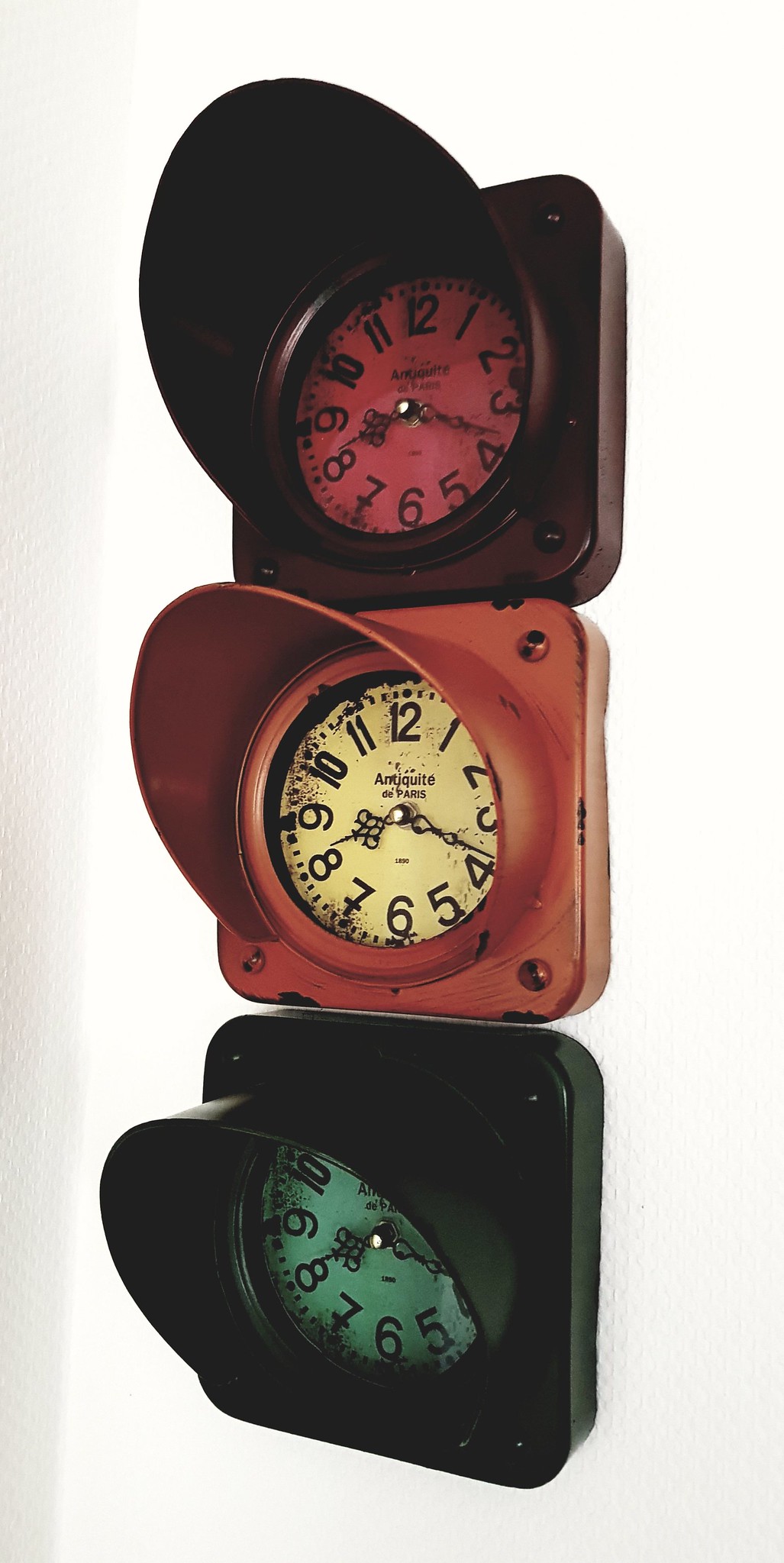This photograph captures a vintage-inspired piece of home decor resembling a traffic signal, cleverly repurposed with clocks instead of lights. The structure mimics a streetlight frame with a top section in dark brown, a middle section in orange, and a bottom section in dark green or black. Each section features a square clock face corresponding to typical traffic light colors: the top is red, the middle orange, and the bottom green. The clock faces are adorned with ornate hands indicating 8:18, and each face prominently displays the text "Antiquité de Paris." The design exudes a shabby-chic aesthetic, with noticeable wear and tear, especially on the middle clock, adding to its antique charm. The edges show signs of wear, and the overall look is slightly dusty and worn, enhancing its vintage appeal. This decorative piece would perfectly complement a rustic kitchen or an industrial loft.